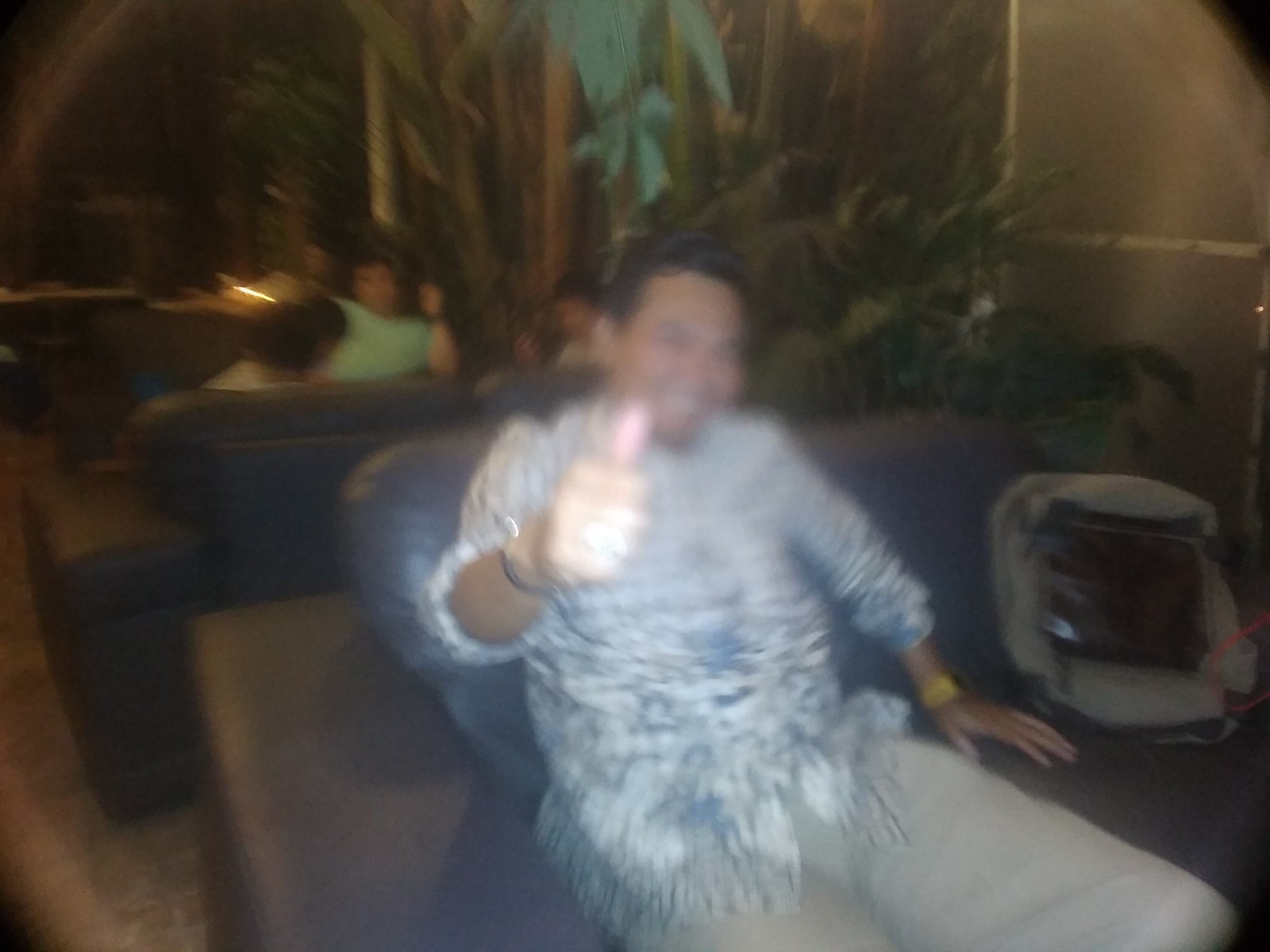In this blurry circular image, likely obscured by a dirty or hazy camera lens, a smiling Asian man wearing a white and black shirt is giving a thumbs up to the camera. The details of his face are indistinct due to the poor image quality. He sports a bracelet on his raised hand and a yellow watch on the other, which rests on the couch beside him. He is dressed in beige pants, and next to him is a backpack. Behind him, a large tropical plant adds greenery to the setting. The background reveals another couch on which four people are seated, one of whom is wearing a green shirt. Further back, there is another couch, a table, and several more plants to the right, enriching the environment with a lush, indoor feel.